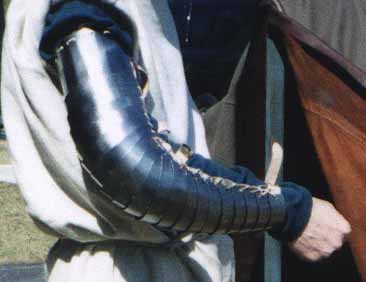The image portrays a close-up of a person's right arm clad in elaborate, Renaissance-style attire. The arm is encased in shiny black leather with an overlaid white or gray tunic, which is subtly detailed with a black ruffled shoulder. Strikingly, the arm features circular discs running up to what appears to be steel sleeve armor, adding a touch of medieval craftsmanship. A white hand emerges from the end of the armor, indicating the individual is white. The scene captures the essence of a knight adorned in knightly armor, possibly beside a horse, with the grass and a black border visible in the bottom left corner, suggesting an outdoor setting.